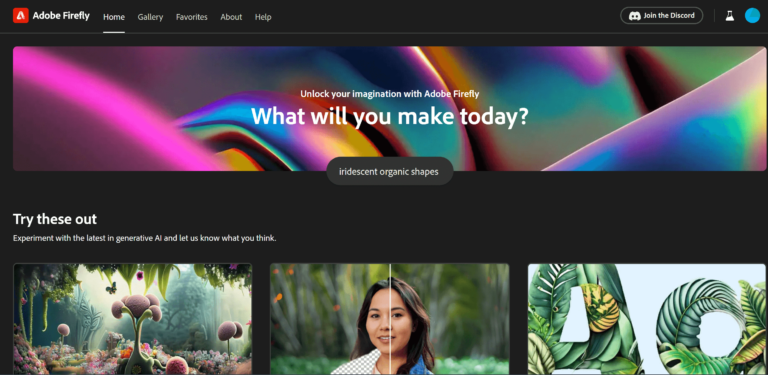In this detailed image from the Adobe Firefly website, the top-left corner prominently features the website's name "Adobe Firefly" next to its logo—a red square containing a white, stylized 'A'. Adjacent to this, a navigation bar displays several categories: "Home" (currently selected and underlined in white), "Has Followed," "Gallery," "Favorites," "About," and "Help."

At the top-right corner, there's a small blue circle icon next to a vial icon, which is next to a speech bubble containing the words "Join the Discord" alongside the Discord logo.

Centrally displayed is a rectangular banner that reads, "Unlock your imagination with Adobe Firefly. What will you make today?" This banner features a colorful, abstract background blending hues of pink, blue, yellow, and red.

Towards the bottom-left of the image, the text "Try these out" introduces three large images. The first, located at the bottom-left, depicts various plants, while the bottom-middle image presumably shows a person.